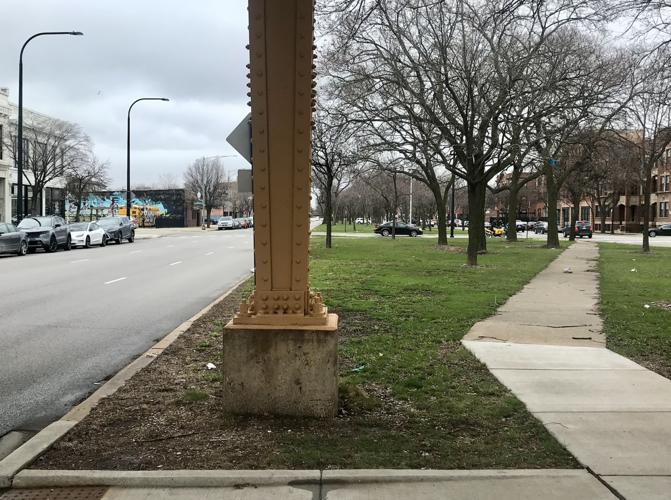This photograph captures a detailed scene of an overcast city street front and center, dominated by a large, riveted, yellow steel pillar mounted on a square cement base held down by massive bolts. To the left, the street, lined with a variety of parked cars and illuminated by streetlights, cuts through the urban landscape, while in the far distance, a train is noticeable. The right side features a footpath with large cement pavers running parallel to a grassy area, interspersed with barren trees, indicative of winter. Further to the right, a sidewalk extends under and in front of these trees and grassy patches. The sky, heavy with clouds, suggests the likelihood of rain. The setting includes various buildings visible at the distance on both the left and right sides, with a white building prominent on the left and others further back by the trees. Additionally, a graffiti wall can be spotted along the far left side, adding an urban character to the scene.